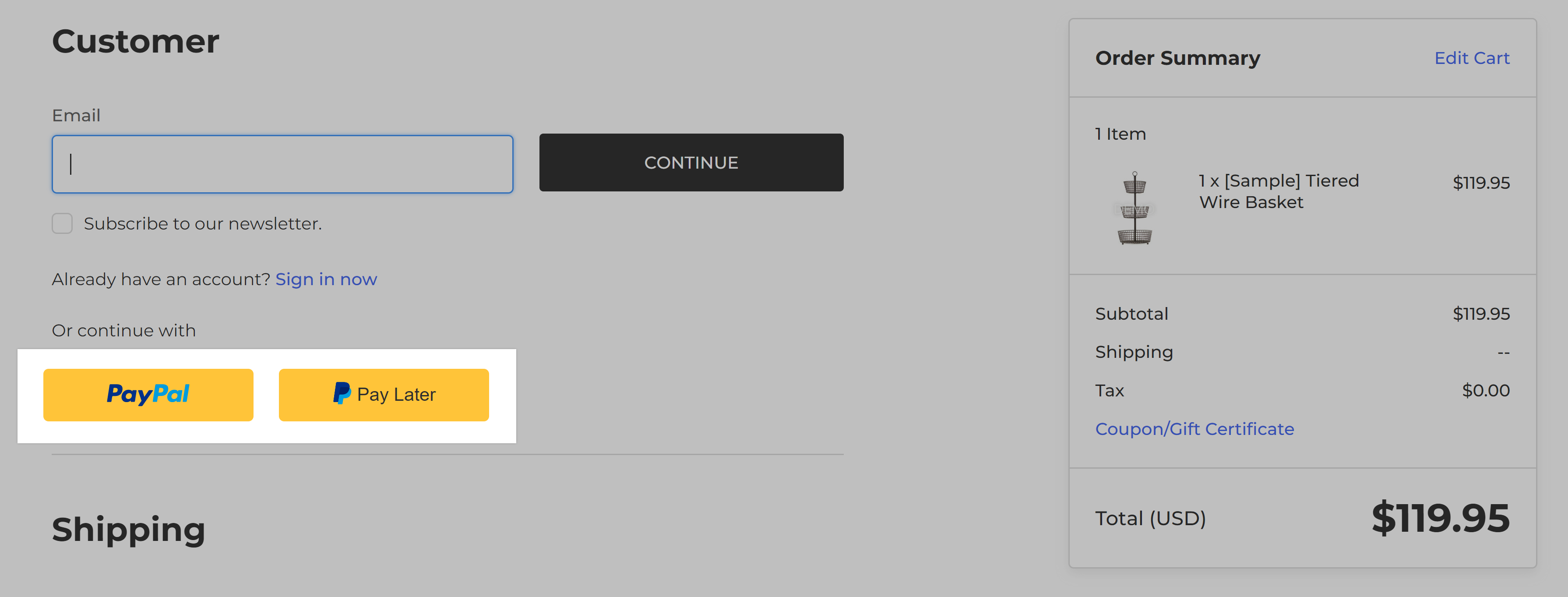Detailed Caption:

The image depicts an online form with a medium gray background, designed for newsletter subscription and purchasing a product. The form includes a prominent email field followed by a large black button labeled "Continue." Adjacent to this is a section labeled 'Order Summary,' detailing the purchase of a "One-Time Sample Tiered Wire Basket" priced at $119.95. The subtotal and total are both listed as $119.95, with no additional shipping costs or taxes. Below the email field, there are multiple interactive elements such as a checkbox for "Already have an account? Sign in now," and options to "Continue with PayPal" or "Pay Later." The PayPal buttons are distinctive, colored in yellow with blue text, and each is encased in a white rectangle, contrasting the overall gray background. The page's color scheme primarily includes shades of gray, black, blue, yellow, and white, creating a clean and user-friendly interface designed to facilitate both newsletter subscriptions and product purchases.